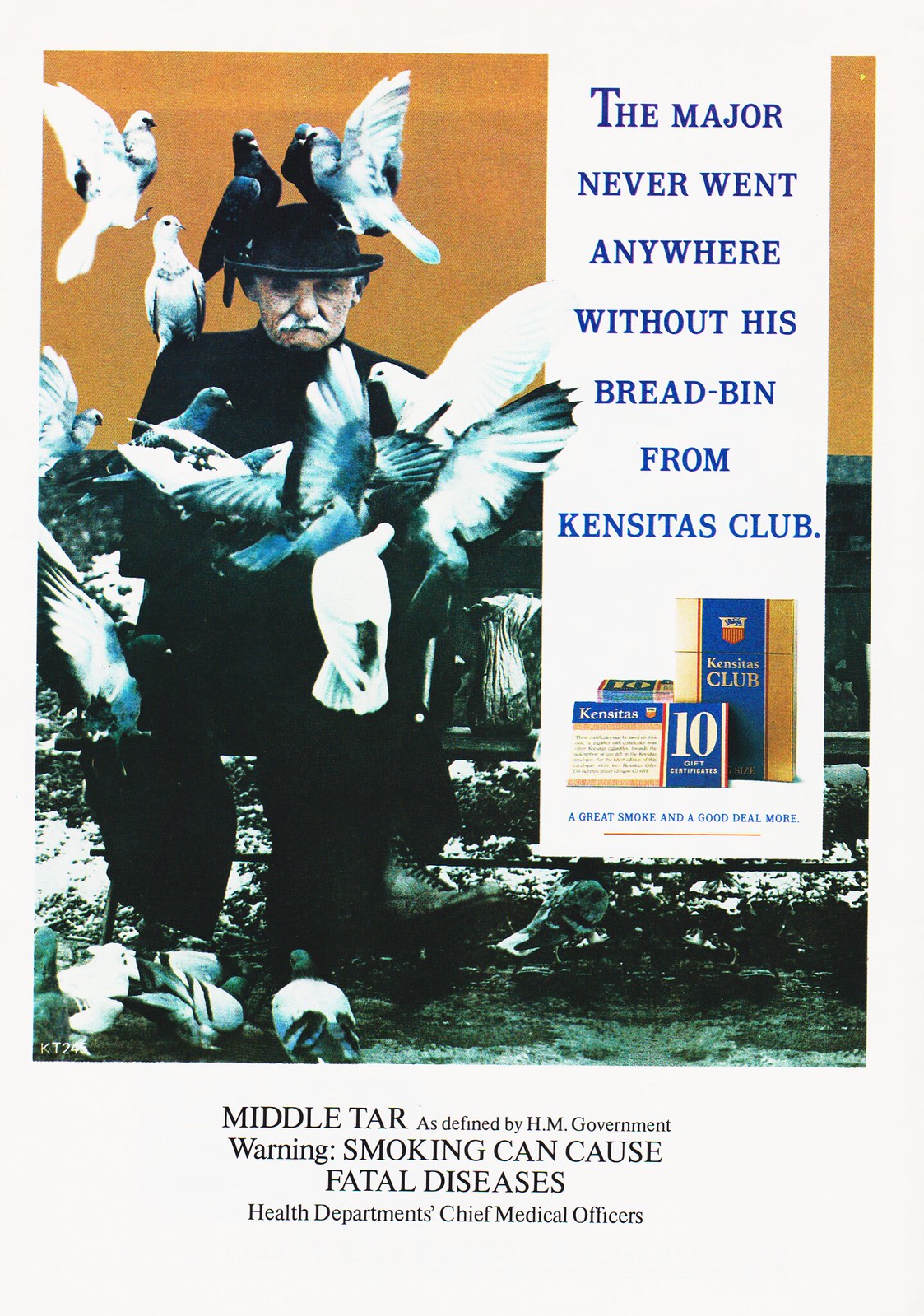The image is an old advertisement poster for cigarettes. The primary focus is on an elderly man with a mustache, wearing a black hat, coat, and pants, seated on a bench. He is covered in pigeons—approximately ten in total—with some perched on his hat and shoulders, others on his lap, and one in mid-flight. The setting is snowy, suggesting a cold environment. To the right of the man, there's a vertical strip of text featuring a humorous advertisement stating, "The Major never went anywhere without his bread bin from Cancita's Club," accompanied by images of two cigarette packs. Below the text, in bold black letters, appears a health warning: "Middle Tar, as defined by H.M. Government. Warning, smoking can cause fatal diseases - Health Department, Chief Medical Officers." The color palette of the poster includes tan, blue, orange, different shades of gray, black, and brown, which gives it a vintage feel.